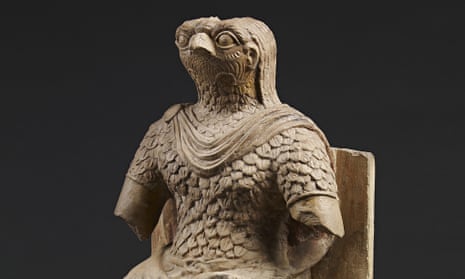The image features a close-up photograph of a wooden statue set against a completely black background. The statue, carved from tan brown wood, presents a unique hybrid appearance, combining features of a human and a bird. The face resembles that of an owl with a wide, round head, prominent white eyes, and a distinct beak situated on a nose that also has a hint of extraterrestrial characteristics akin to E.T. The statue's human-like torso is adorned with what appears to be a feathered or scaly pattern and is draped in a cape or scarf extending over its shoulders. Notably, both arms of the statue are cut off just before the elbows, creating a truncated appearance. The figure seems to be seated, possibly on a chair, with a wall faintly discernible behind it. The statue also has slicked-back hair flowing down to its thick neck and shoulders, enhancing its enigmatic and mythical aura.